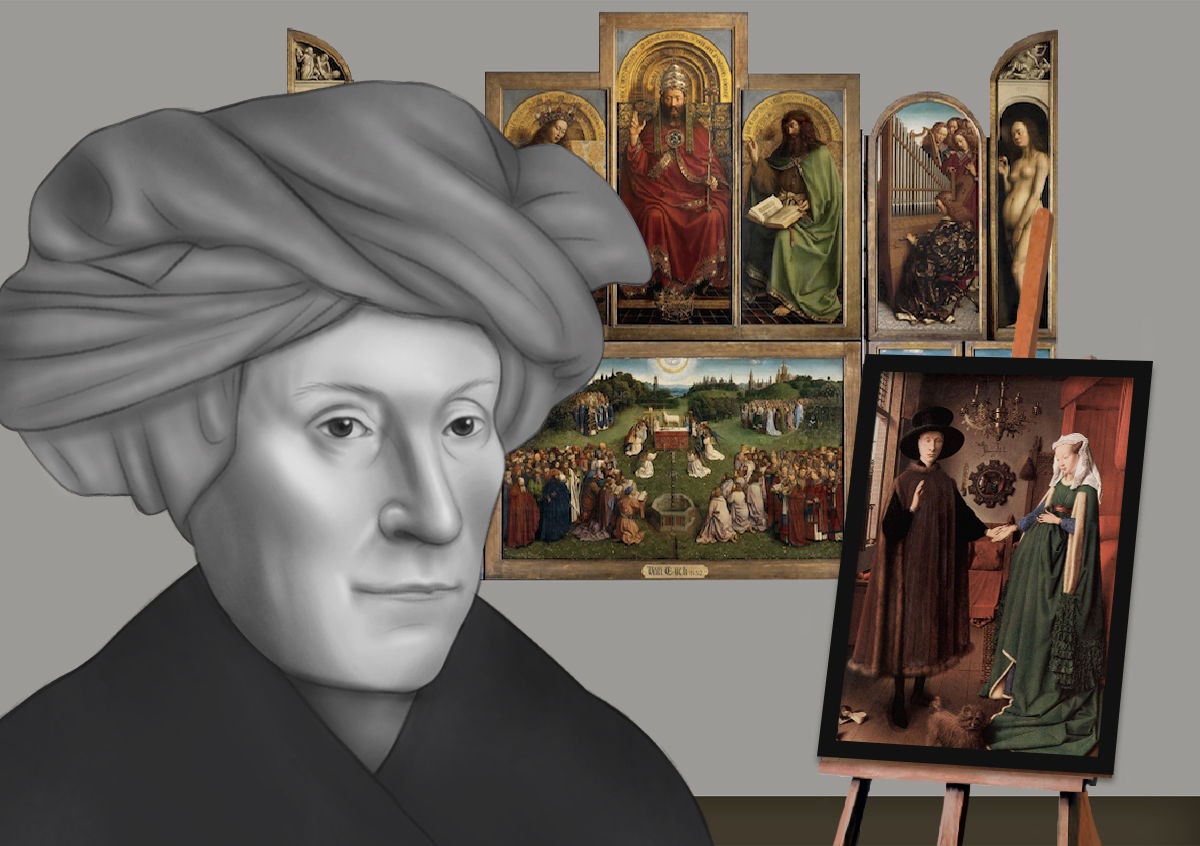The rectangular digital artwork features a black and white depiction of an older woman, visible from the shoulders up and positioned on the left side of the image. She is wearing a simple black garment and a gray headscarf, with her head tilted diagonally to the right. This monochrome figure contrasts strikingly against the background, which showcases a gray wall adorned with numerous old-fashioned and religious paintings in golden or brown frames. These colorful paintings include a variety of subjects: a royal figure flanked by two individuals, a pregnant nude woman, a woman playing a harp, and other historic or religious iconography. Additionally, a distinct painting displayed on an easel to the right features a man and woman holding hands with a small dog at their feet, dressed in an old-fashioned manner. The wall and the ground beneath emphasize the classical ambiance, tying the elements of the artwork together in a cohesive yet intricate scene.